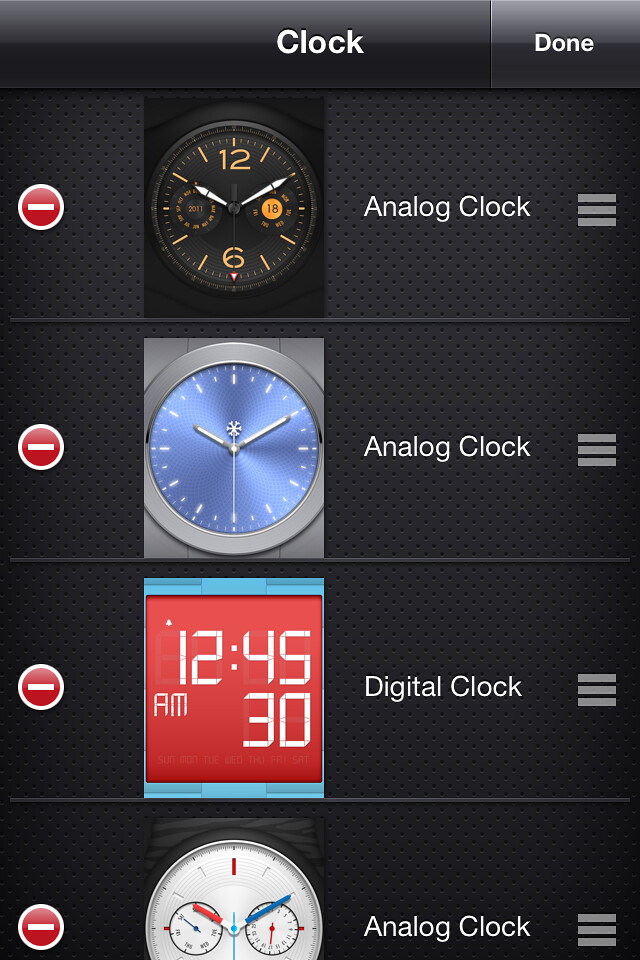The image displays a clock selection screen set against a black background. At the top, the word "Clock" appears in white letters, with a "Done" button to the right encased in a gray background also with white text. Below, there are four different options for clock faces, each within a textured gray and black pattern background:

1. **First Clock (Topmost)**: This clock has a dark face with orange numbers for 12 and 6, while the rest are indicated by white marks. It features white hour and minute hands, with the latter positioned at what appears to be 10 o'clock, suggesting a time of 10:30 AM or PM, as the second hand points at the 6 (30 seconds). There are two small circular dials below, likely displaying the year and day. To the right, labeled in white letters, it says "Analog Clock." This option has three rectangular lines symbolizing settings.

2. **Second Clock**: A circular gray clock with a blue face and white markings for hours and minutes. The clock face is well-lit, with the second hand featuring a snowflake-like design at one end and pointing towards 30 seconds. The hour hand points at 10 and the minute hand at 2, indicating a time of 10:10 AM or PM. Also labeled "Analog Clock" in white letters, this option includes the same three rectangular lines for settings.

3. **Third Clock**: This is a red square clock face with digital white numbers displaying "12:45" and "AM" beneath it. Below the time, the number "30" suggests the date. The red clock face has a blue outline, and it is labeled "Digital Clock" to the right.

4. **Fourth Clock**: This is another round clock with a white face, a red tick at the top, and gray lines marking the minutes. It lacks numerical hour markers. It features three hands: a blue minute hand, a bright blue second hand, and a red hour hand. It is labeled "Analog Clock" to the right. Two small circular clocks are present within the main face, though their details are indistinct. Each clock choice has a red circle with a white outline and a white dash to the left. 

This detailed description captures the essence and specifics of each clock face option within the selection screen.